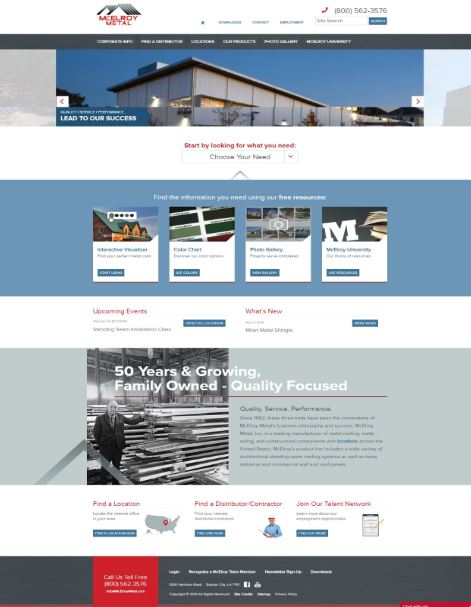The screenshot showcases the homepage of a website advertising metal sidings, likely used for building exteriors. At the top of the page, the company's name, "Meldorot," is displayed, albeit not very clearly. Accompanying the name is a logo with red lettering and a prominently placed telephone number for customer inquiries.

The page layout is divided into well-organized sections. The header features a slideshow gallery of various building exteriors, navigable via arrows on either side. Below the header, a search box invites users to "start by looking for what you need" with options to choose specific requirements.

Following the search section, there are clickable images that appear to link to stories or blog posts. Just beneath this, a prominent section highlights the company's long-standing history with the caption "50 years and growing, family owned, quality focused." This segment includes a nostalgic black-and-white photograph of an elderly gentleman, possibly from the 1950s or 1960s, standing next to a stack of what seems to be wooden or metal planks.

Further down, another section offers practical tools for visitors, including links to "find a location," "find a contractor," and "join our network." The footer of the page is predominantly dark grey, accented with red edging, featuring white and red text to ensure legibility against the dark background.

Overall, the webpage effectively communicates the offerings and heritage of this metal siding manufacturing company, reflecting both its products and commitment to quality.